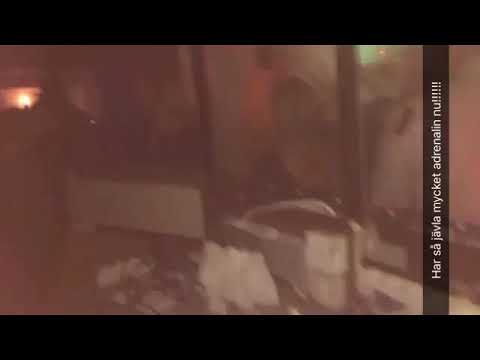This image depicts a chaotic outdoor scene, possibly the aftermath of a significant event such as an earthquake or an intrusion. The picture is very blurry, with visible signs of destruction, including rubble and what may be a cracked storefront window. There are black borders framing the top and bottom of the image and text running vertically along the right side, rotated counterclockwise. The text, appearing to spell "H-A-R S-A J-A-V-A-L-A M-Y-C-K-E-T A-D-R-E-N-A-L-I-N N-U!" with multiple exclamation points, is mostly in white font. While the exact meaning of the text is unclear, it may suggest a heightened state of emergency or excitement. There's a faint light in the top left corner, possibly from a patio light, and blurry figures can be seen through what appears to be a window, hinting at the presence of people in a building. The scene is dark with hints of greenery and a sense of urgency or distress is evident throughout the composition.